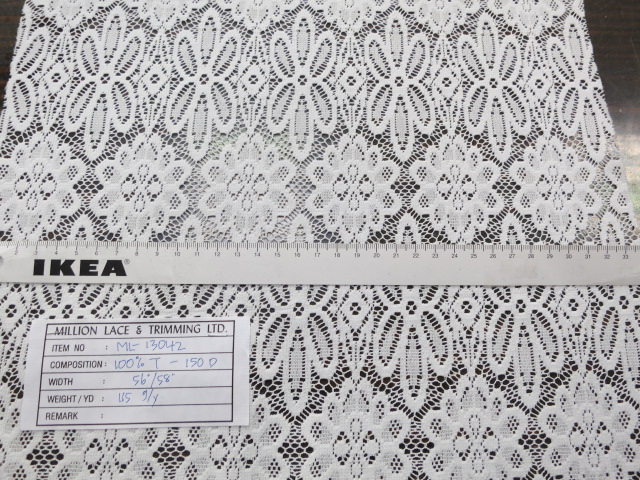The image depicts a delicate white lace sample featuring intricate floral patterns, where the top pattern shows flowers with large petals and the subsequent one showcases flowers with many more petals and four circles at the center. The setting appears to be in an IKEA store, as indicated by the white tape measure with black lettering and numbering, reading "IKEA" and spanning from 1cm to 33.5cm. Draped over the lace, the tape measure partially covers a tag in the lower left, which is black and white and handwritten in blue ink. The tag reads "Million Lace and Trimming LTD," with item number ML-13042, composition 100% T-150D, width 56cm x 58cm, weight 115 yards, and a section marked "Remarks." The lace, entirely white, is presented on a clean, flat surface, highlighting its intricate design and craftsmanship.